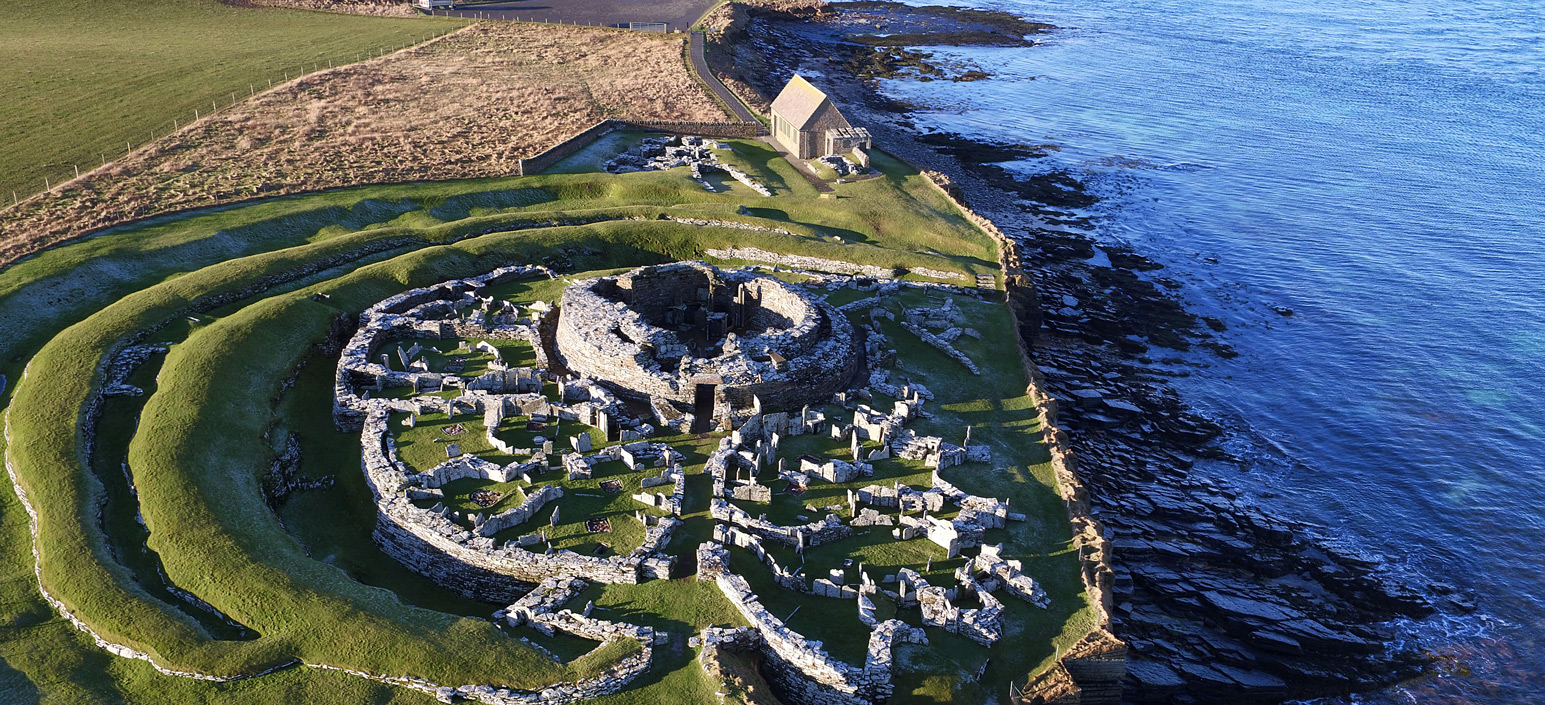The image is an aerial photograph of a coastal island, likely in the UK, viewed from approximately 600 meters above. Dominating the scene are lush, rolling hills blanketed in vibrant green grass. In the foreground, the coastline divides the image with the tumultuous sea on the right and the verdant land on the left. Central to the landscape is a complex, ancient ruin that resembles a fort. This circular structure, composed of white stone, displays zigzagging stonework and multiple concentric rings of stones, reminiscent of Stonehenge, though partially in ruins. Adjacent to these ancient structures are smaller, open stone areas, which also exhibit signs of age and overgrowth. In the background, slightly distant from the ruins, stands a modest house, possibly hinting at a golf course nearby. The composition and elements strongly suggest a picturesque, historical site nestled in an island nation like the United Kingdom.